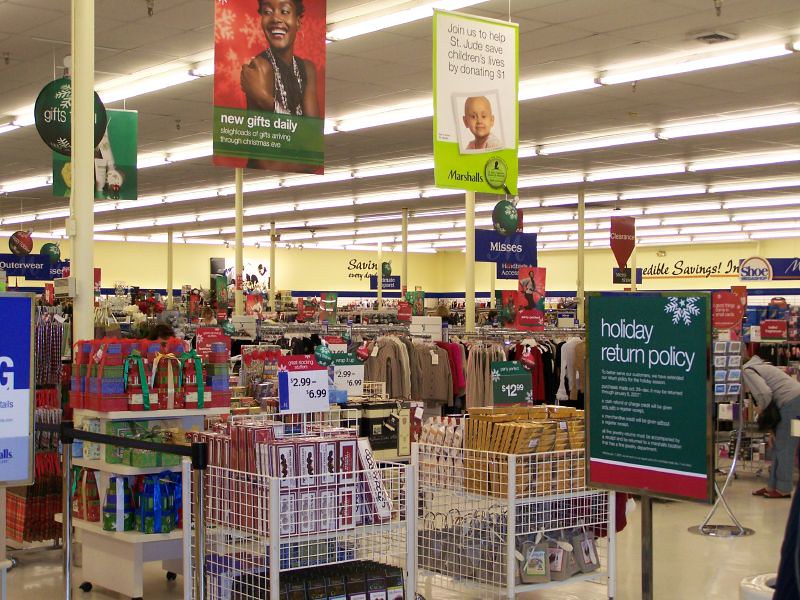The image captures the bustling interior of a Marshall's department store during the holiday season. Prominently displayed is a sign about St. Jude's, hanging from the ceiling, indicating the store's support for the children's research hospital. A nearby poster features a smiling Black woman and the phrase "New Daily Gifts," highlighting the store's frequent arrival of new merchandise.

In the foreground, a shopper dressed casually in jeans and a gray sweatshirt examines the array of holiday items. The store is decorated in festive reds and greens, with various bins filled with products designed to attract holiday shoppers. An "Incredible Savings" sign is displayed on a yellow side wall, a signature message of Marshall's promise of value deals.

The image shows the store's bright atmosphere, illuminated by numerous fluorescent lights lining the ceiling. Sweaters, gift bags, and other seasonal items are neatly arranged for easy browsing. In the distance, the housewares section of the store is visible, indicating the store's expansive layout. The overall impression is one of a well-stocked, inviting department store, bustling with holiday shoppers and festive cheer.